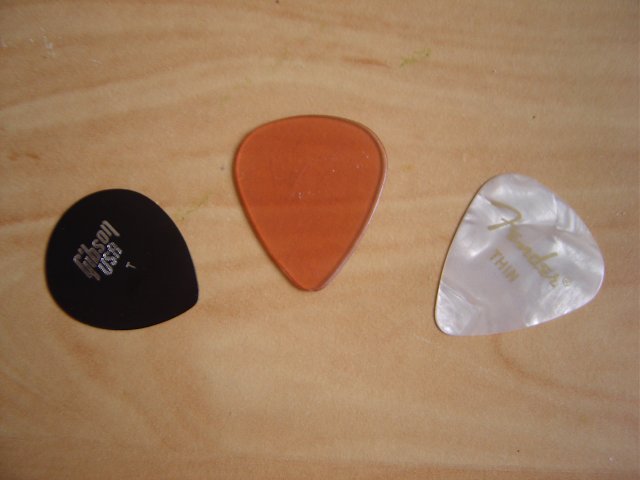This photograph showcases a trio of guitar picks meticulously arranged on a light brown, wood-grain table. The table, reminiscent of a rich beige brownie hue, features darker grain lines running through it, providing a natural and textured backdrop. 

On the left is a black guitar pick that appears worn and slightly faded. It prominently features the brand name "Gibson" in gray letters, along with "USA" and the letter "T" in white, denoting its origin and thickness. 

The center pick is a simple, unadorned piece of a brownie-orange color, with a slightly darker border, giving it a minimalist yet distinct appearance.

On the right rests the third pick, distinguished by its white, marble-like texture. Although some text is partially illegible, the word "THIN" can be discerned, indicating its type. 

This detailed composition captures the varying colors, textures, and branding details of each pick, set against the beautifully patterned table surface.